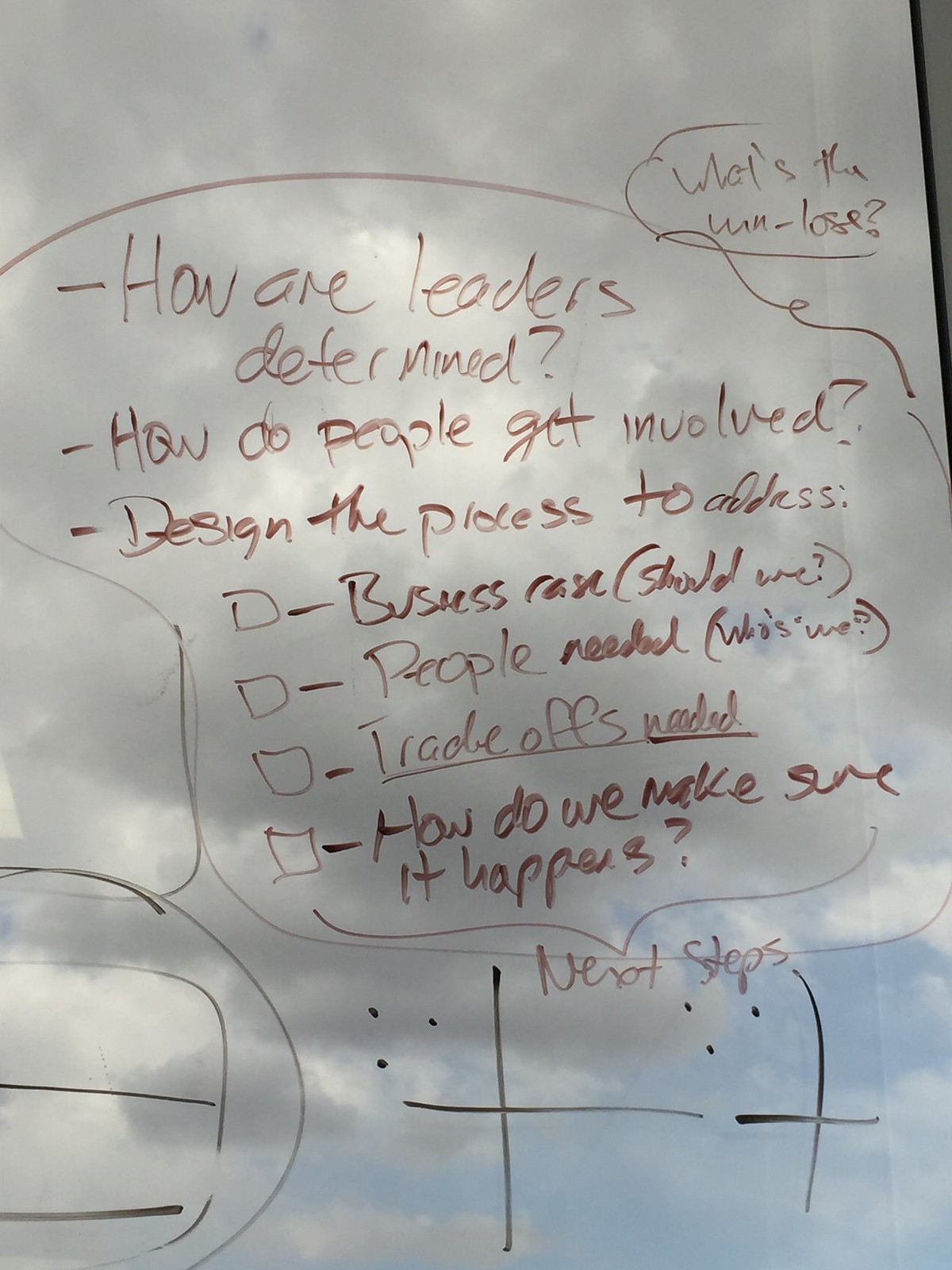The image is a color photograph in portrait orientation featuring a white document with handwritten notes in brown marker, likely intended for a classroom-style presentation. The top right corner contains a half circle enclosing the question, "What's the win-lose?" Directly beneath this are a series of bullet points addressing various aspects of a leadership process: "How are leaders determined?" "How do people get involved?" and "Design the process to address:". Following this are sub-bullets indicating key considerations such as "Business case (should we?)", "People needed (who's we?)", "Trade-offs needed", and "How do we make sure it happens?" A curly brace leads from these points to the concluding note, "Next steps." The document also features visual elements like grids or cross symbols with plotted dots, set against a backdrop that includes mostly gray clouds with some white and hints of blue sky.